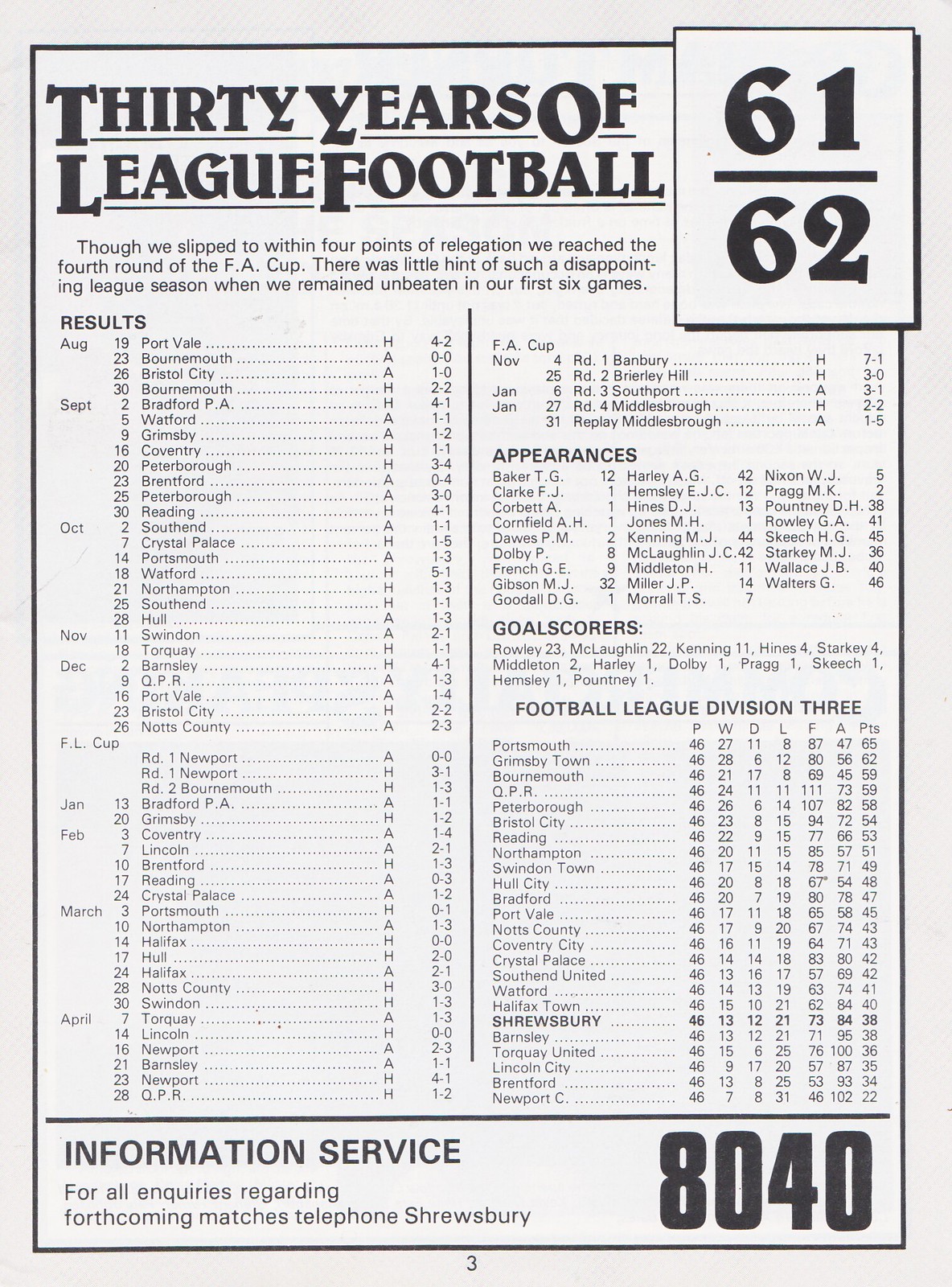This is an image of an informational sheet entitled "30 Years of League Football" in black text at the top left corner. Adjacent to it on the top right is "61" followed by a horizontal line and then "62," likely indicating the 1961-62 season. The sheet is divided into two columns. The left column starts with a paragraph that includes, "Though we slipped to within four points of relegation, we reached the fourth round of the F.A. Cup. There was little hint of such a disappointing league season when we remained unbeaten in our first six games." Below this paragraph is a section labeled "Results," listing dates, teams, matches, and scores of English soccer matches. The right column contains three sections: "Appearances," "Goalscorers," and "Football League Division 3," which likely include player stats and league standings. The entire sheet is in black and white, with a white background and black text. An advertisement is featured at the bottom of the page.